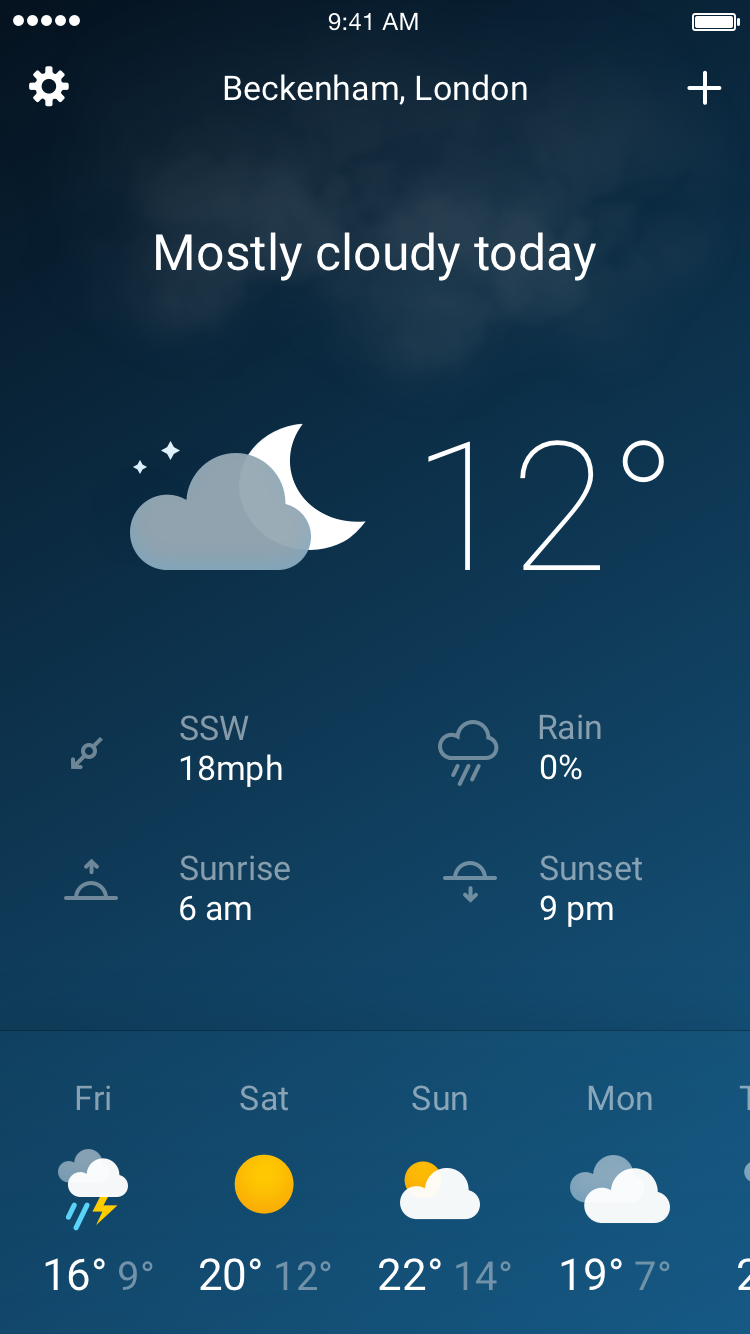This is a detailed screenshot of a weather app displayed on a smartphone. The background transitions from dark blue at the top, with a few white clouds, to a lighter blue downwards.

**Top Section:**
- The top left corner features three white horizontal dots.
- In the center, the time is displayed as "9:41 AM" in white.
- The top right corner shows a full battery icon with a small white plus sign beneath it.

**Main Display:**
- The location is identified as "Beckenham, London" in white text.
- Below the settings gear icon on the left, the text "Mostly cloudy today" appears in the middle.
  
**Weather Icons and Information:**
- To the left, a cloud overlaps the right side of a half-moon with two stars to the left of the cloud, showing the current conditions as "12°C."
- Under the cloud, it says "SSW 18 mph," indicating the wind direction and speed.
- To the left of this wind information, an arrow pointing down and left with a gray circle in the center further details wind direction.
- To the right, a cloud icon with rain droplets indicates "Rain 0%," suggesting no expected precipitation.
- Beneath the arrow, there is a sun partially obscured by a line and an arrow pointing up, symbolizing sunrise at "6 AM."
- Similarly, the sunset is indicated at "9 PM" on the right side of the sun display.

**Forecast Section:**
- The bottom section displays a four-day weather forecast, encompassing Friday through Monday, from left to right.

This detailed layout provides a thorough synopsis of the current weather conditions and upcoming forecast for Beckenham, London, ensuring clarity and ease of understanding for the viewer.